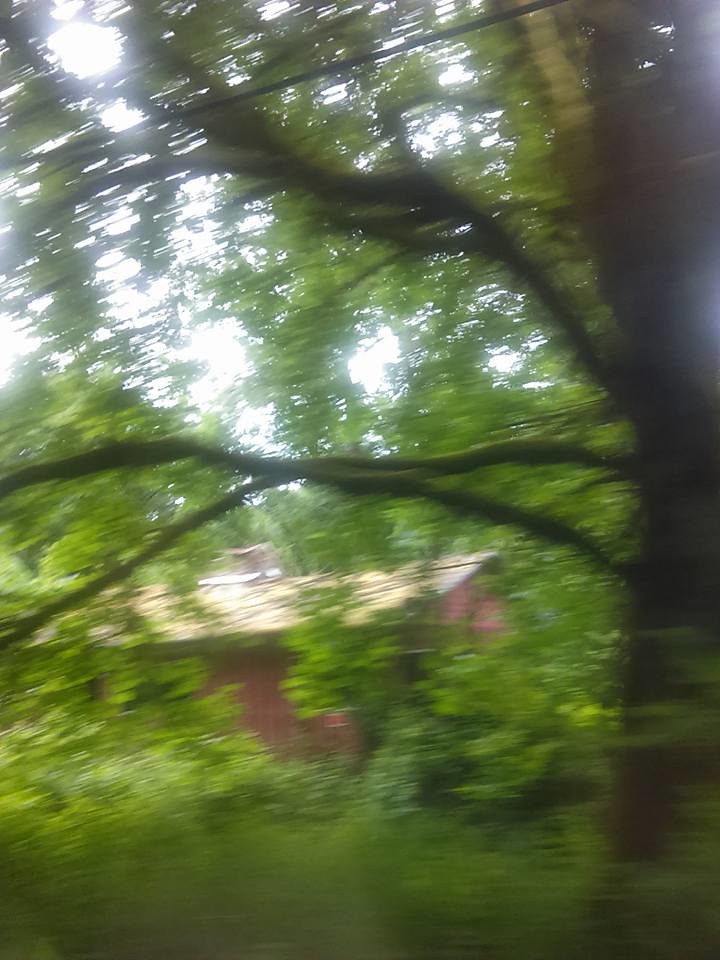A picturesque scene depicts a classic red barn nestled in a remote and tranquil environment, likely on a farm. The foreground is dominated by an array of lush, verdant trees, amongst which stands one particularly large brown tree with extensive, sweeping branches. The barn, accented with a chimney or possibly an additional small structure on top, is surrounded by ample green space, epitomizing a serene and peaceful setting. Bathed in daylight, with the sun casting a partial glow, the area exudes summertime charm, evident from the trees fully adorned with leaves.